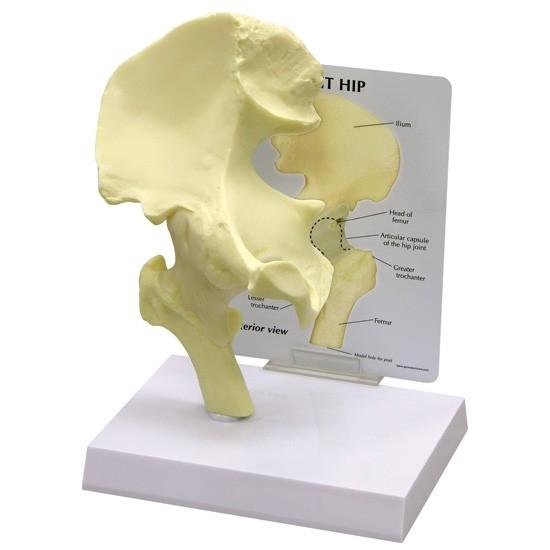This image features a highly detailed, color model of a human hip joint, mounted on a marble-like white base. The hip model, which is almond or off-white in color, displays the intricate structures of the hip, such as the ilium, head of femur, and articular capsule of the hip joint. The backdrop consists of a white card, held in place by a piece of plastic at the bottom, which provides a comprehensive diagram of the hip, labeling and mapping the various parts to correspond with the 3D model. This educational setup, reminiscent of what might be found in a doctor's office or an anatomy class, facilitates a clear understanding of the hip's anatomy through its meticulously labeled and depicted elements.